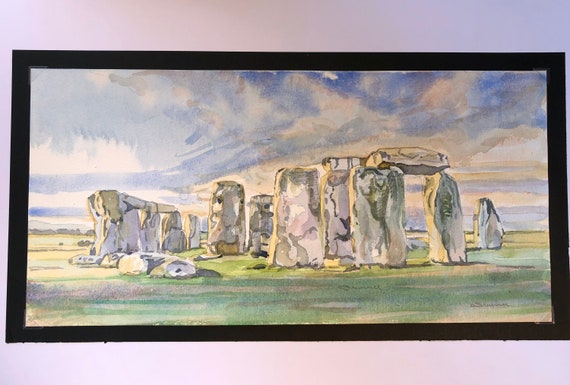The image displays a watercolor painting of Stonehenge in England, encased in a black frame and hung on a white wall. The composition features Stonehenge prominently in the center, with its characteristic grey stones depicted in a slightly rough and undetailed manner, adding an abstract quality to the artwork. Surrounding the ancient structure are green grass fields, illustrated with varying shades including hints of yellow and blue. The sky above is a mixture of vibrant blues with white, fluffy clouds scattered throughout, complemented by subtle touches of orange suggesting early morning or late afternoon light. The watercolor technique, evident from the softly blended colors, imparts a somewhat muted and dreamy atmosphere to the scene. Near the bottom right corner, there appears to be an indistinct signature of the artist. The overall effect is a serene and artistic representation of one of England's most iconic landmarks.